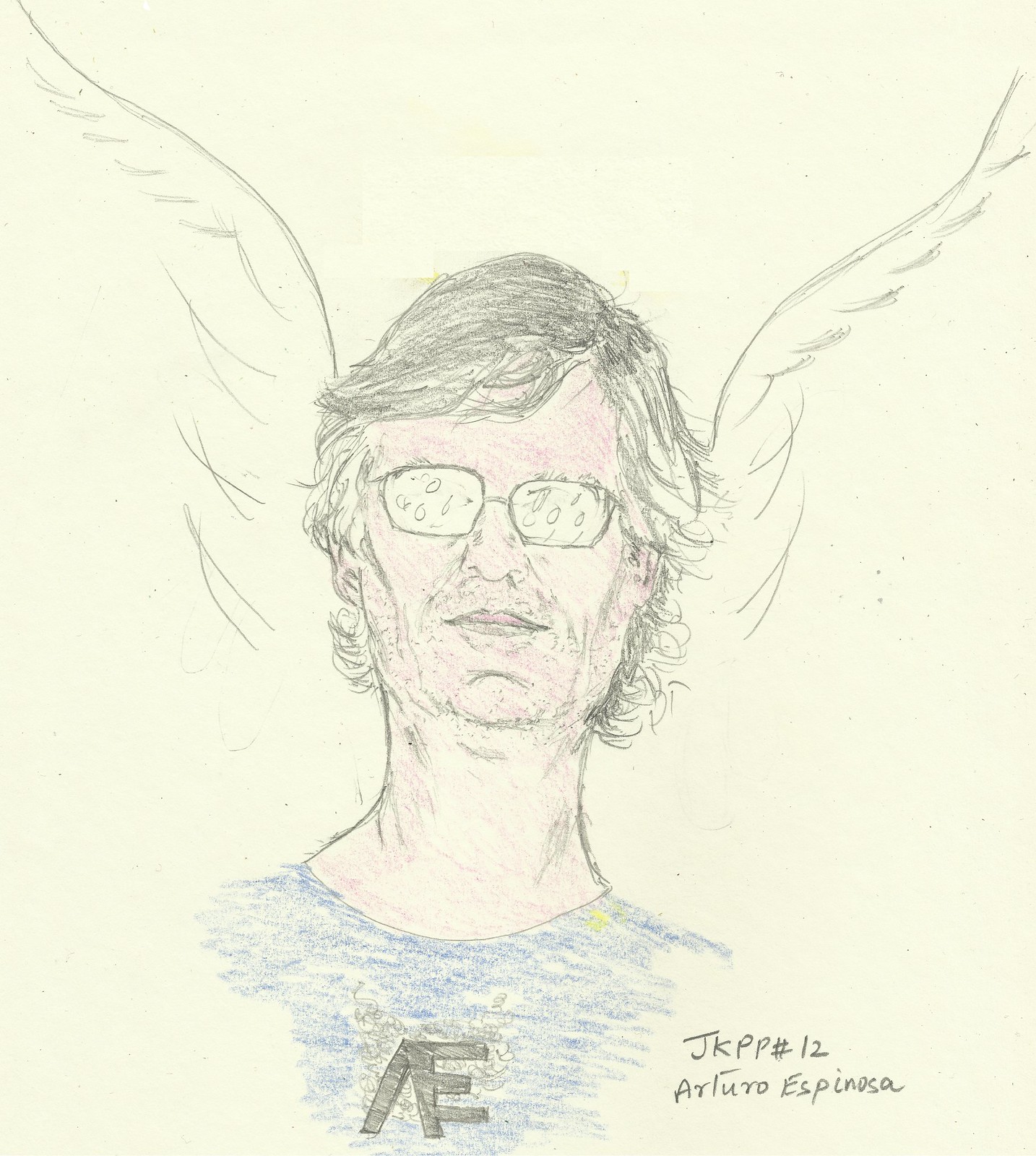This image is a detailed color pencil sketch in a landscape orientation, featuring the head and shoulders of an adult man, likely between 25 and 40 years old. The man, appearing Caucasian with a peach or pink skin tone, has longish, shaggy, dark hair that is wavy and feathered around his ears and extending to his neck. He has some facial hair and is wearing dark-rimmed glasses, through which his eyes are not clearly visible. A blue t-shirt, lightly colored and featuring intertwined letters "AE" on the front, covers his lean and visible long neck. The man holds a neutral or slightly smiling expression, with a subtle reflection of droplets of water visible in his glasses. Lightly sketched, large angel wings emerge symmetrically from behind his head, perhaps as a tribute to someone. The artwork bears the signature “JKPP number 12 Arturo Espinosa” in the bottom right corner.